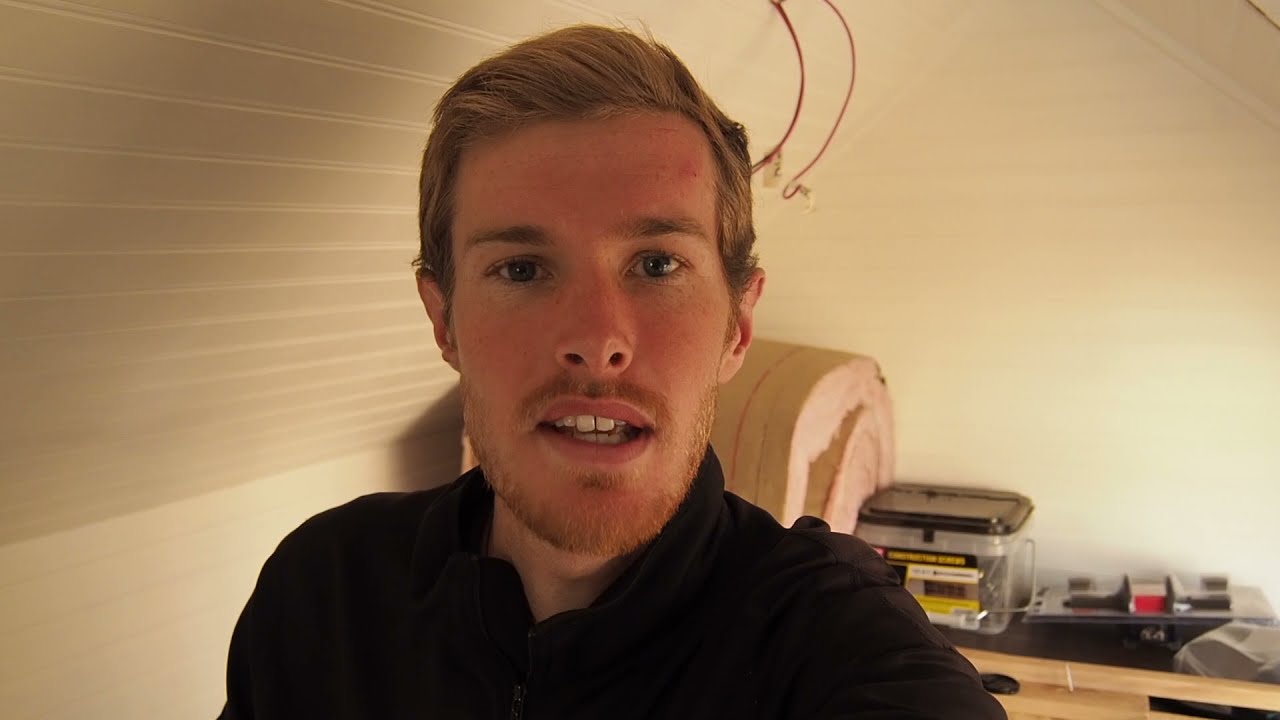The image features a young, white male, possibly in his mid to late 20s, with blonde hair that is parted on the left and styled back, and a short beard and mustache that match his hair color. He is wearing a dark, button-down collared shirt which may be long or short-sleeved. He appears to be taking a selfie or a screenshot from a selfie video, and his mouth is open as if he is speaking, giving an awkward smile. The setting resembles an attic or workshop-like room with sloped white wood-paneled walls and a white ceiling. Behind him, there is a desk cluttered with various items including containers with yellow and black writing, plastic items, and a possible piece of wood, along with electrical wires and a red wire hanging down from the ceiling.